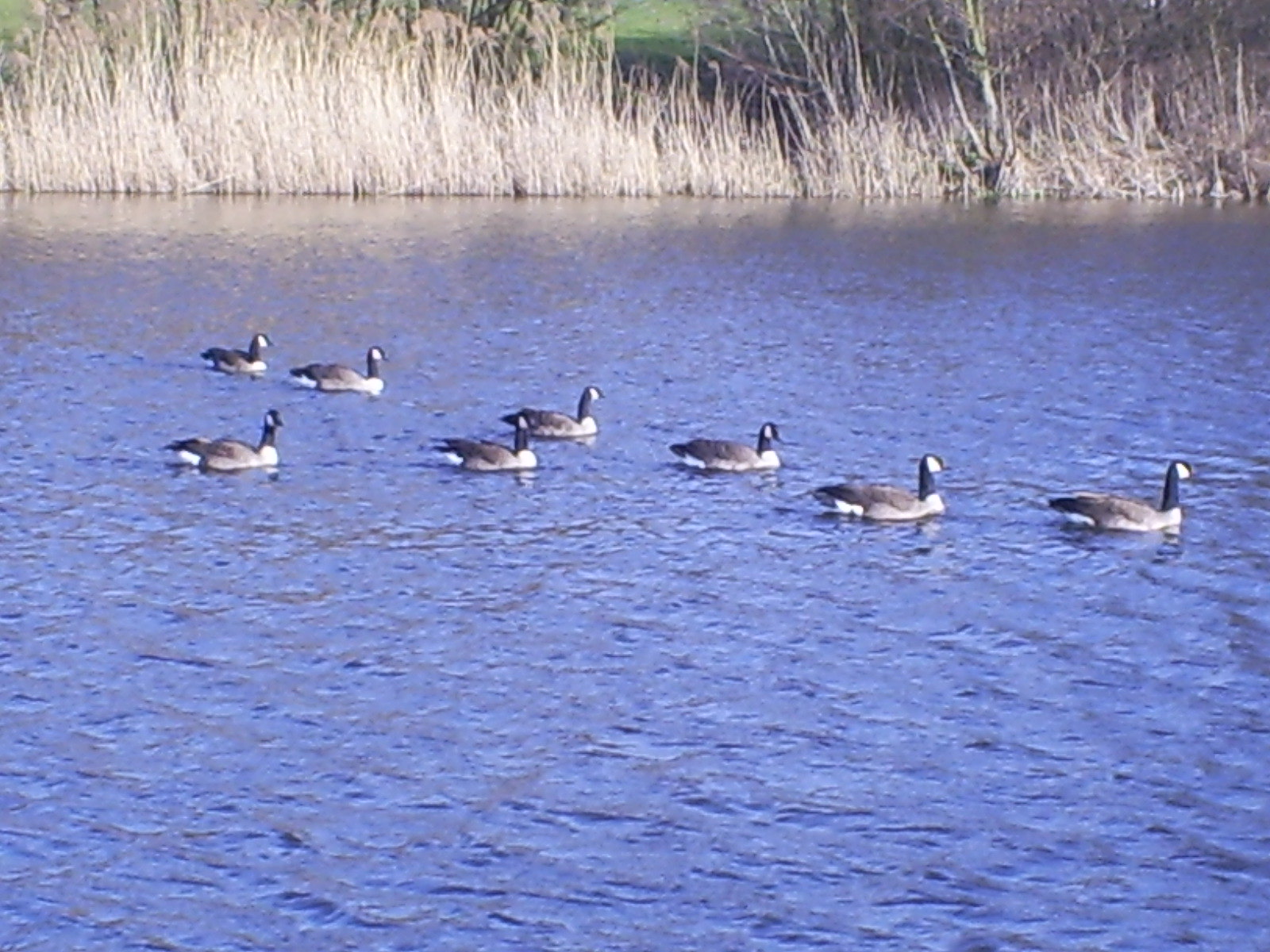This color photograph, likely taken from the shore or a boat, captures a serene outdoor scene featuring a group of eight Canada geese swimming in a V formation on a blue lake. The geese are distinctly marked with black necks and white facial patches, complemented by their brownish feathers. The backdrop reveals tall, dying yellowish-beige grass, ascending a hill, with hints of green vegetation further away, suggesting the setting might be a lake, pond, or marsh. Though the image quality is slightly blurry, the natural beauty and tranquil atmosphere are unmistakable, showcasing the geese gracefully gliding on the water's surface under the daylight.